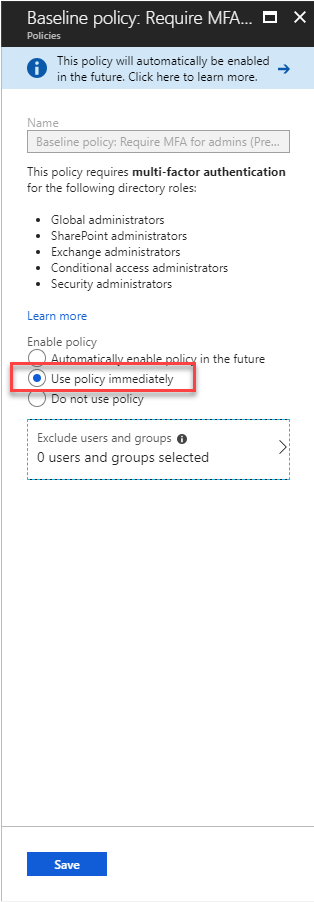This screenshot captures a section of a website dedicated to implementing a policy page. At the top, a header reads "Baseline Policy Require MFA...," though the rest of the text is truncated. Directly beneath this header, a blue bar with an information icon states, "This policy will automatically be enabled in the future. Click here to learn more," accompanied by a right-pointing blue arrow.

Below the blue bar, there is a form section designated for selecting a policy name. Pre-filled text in a grayed-out box displays, "Baseline Policy Require MFA for Admins," indicating that the name is not editable. An explanatory paragraph below this box reads, "This policy requires multi-factor authentication for the following directory roles: Global Administrators, SharePoint Administrators, Exchange Administrators, Conditional Access Administrators, Security Administrators." A "Learn more" hyperlink in blue text follows this description.

Further down, users can enable the policy through three radio button options. The middle option, "Use policy immediately," is pre-selected and highlighted with a red outline. Adjacent to this section, a dotted blue box indicates, "Exclude users and groups," with the current status noting, "0 users and groups selected."

At the very bottom of the interface lies a "Save" button for finalizing and saving the configuration options.